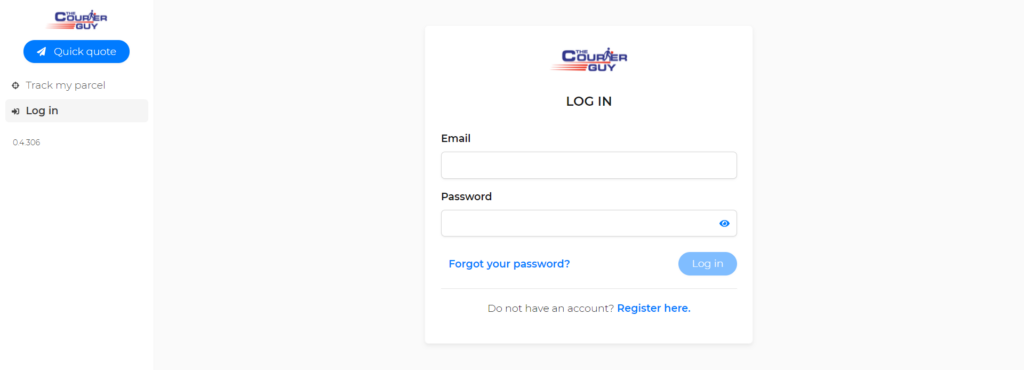The image depicts a section of a web page themed around a service titled "The Career Guy." The layout features a predominantly bluish color scheme with accents of red. A logo, likely representing a person in motion, is visible in the top portion.

On the left side of the page, notable elements include:
- A section prompting users to "Get a Quick Quote," accompanied by a blue clickable button.
- Below this section is an option to "Track My Parcel."
- An area for user login, with an identifier "04306" located just below it.

The central portion of the page showcases a faint gray rectangle that forms the background, overlaid by a white square. The top of the white square prominently displays the title "The Career Guy" and contains a login prompt.

Key features in this central white square include:
- "LOG IN" in bold, uppercase black letters.
- Input fields to enter email and password, labeled "Email" and "Password," respectively.
- A small blue circle next to the password input field.
- A link in blue for users who have forgotten their password: "Forget your password."
- A prompt for new users, stating, "Do not have an account?" followed by a blue "Register here" link.
- A blue "Log In" button at the bottom.

The page design aims to facilitate easy login and account management for users, with a clean and organized layout.